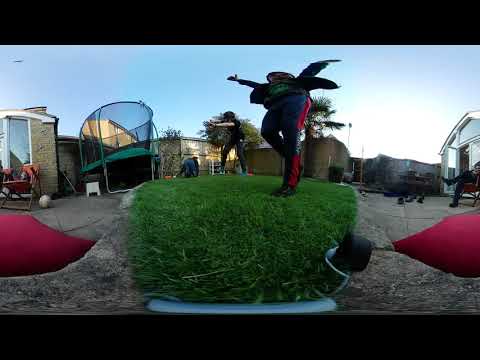The photograph captures a vibrant and slightly distorted scene in a backyard. At the center, a person, likely a child, stands energetically with their arms raised, dressed in dark blue pants accented with red. They are on a lush, green grassy patch, which stands out vividly against the surrounding elements. To either side of the grassy area, there's a brown, possibly artificial ground. The background reveals a mix of structures: a yellow brick house, a glass-enclosed patio, and a shed. Additionally, outdoor elements like a soccer ball, a lawn chair, and a round green trampoline add to the lively setting. The sky above is a clear light blue, and sunlight brightens the scene from the right. Scattered red pieces, resembling rugs or carpets, lie around, and an adult is visible, seated with legs crossed. There appear to be at least three or four people, possibly more, in various areas of the yard. The photograph is horizontally framed with black strips at the top and bottom, suggesting a panoramic or filtered distortion effect.